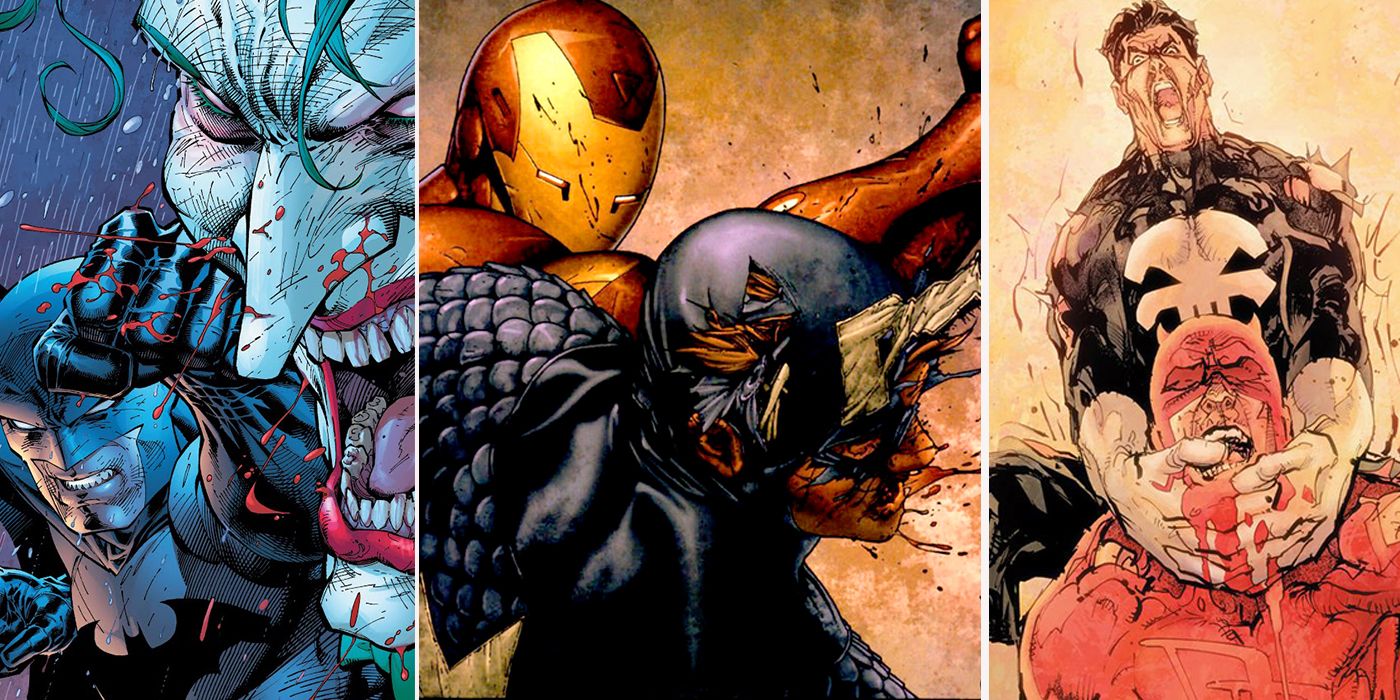This composite image features three distinct comic strip panels, each capturing a dramatic moment of superhero combat. On the far left, a dark and intense scene unfolds as Batman, clad in his iconic dark suit, lands a powerful punch on the Joker's face, causing blood to splatter from the villain's mouth. The Joker's sharp nose, wide red lips, and visible teeth emphasize his twisted delight amidst the violence, all set against a moody blue and black background. The central image spotlights a tense confrontation between Iron Man and Captain America. Iron Man, in his red and gold suit, extends his arm to deliver a punch to Captain America, who stands in the foreground with his head turned to the side, dressed in his blue costume. Blood is visible from the impact, adding to the scene's intensity. The final panel on the right depicts the Punisher, marked by the skull emblem on his chest, as he chokes Daredevil with his black-gloved hands. Daredevil, wearing a red suit, appears to be in agony, with blood dripping from his mouth and hands, heightening the scene's brutal atmosphere. Each panel is a vivid portrayal of conflict, rich in detail and emotion.